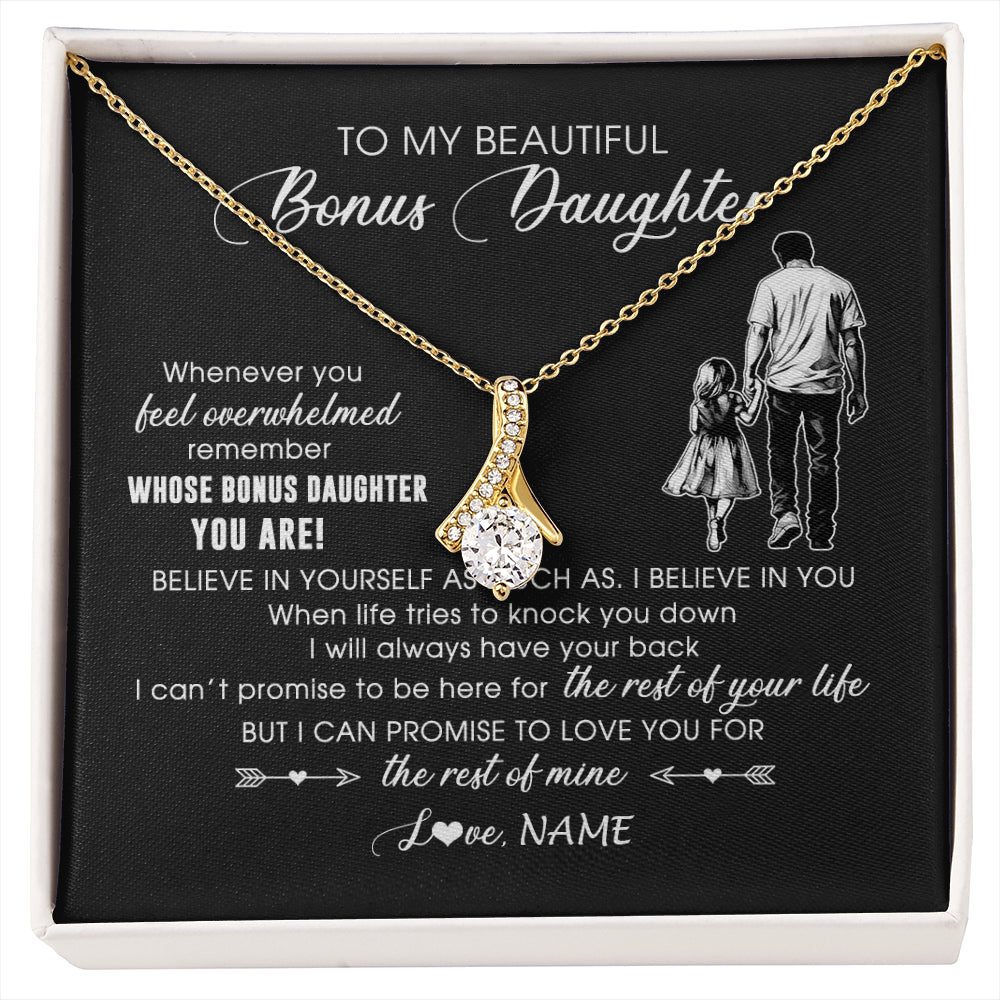The close-up image depicts a piece of jewelry in a white-bordered box, viewed from above so only the box's edges are visible. Inside, the box's background is black and features an emotionally charged message in a mixture of cursive and regular print. The message reads: "To my beautiful bonus daughter, whenever you feel overwhelmed, remember whose bonus daughter you are. Believe in yourself as much as I believe in you. When life tries to knock you down, I will always have your back. I can't promise to be here for the rest of your life, but I can promise to love you for the rest of mine." A gold necklace hangs from the top corners of the box. The necklace forms a V shape and features a slingshot-shaped gold pendant adorned with tiny diamonds that align in a single line, culminating in a large diamond at the center. A poignant illustration accompanying the text showcases a man walking with his daughter, emphasizing the heartfelt nature of the message. This image suggests a personalized, heartfelt gift designed to offer support and unwavering love.